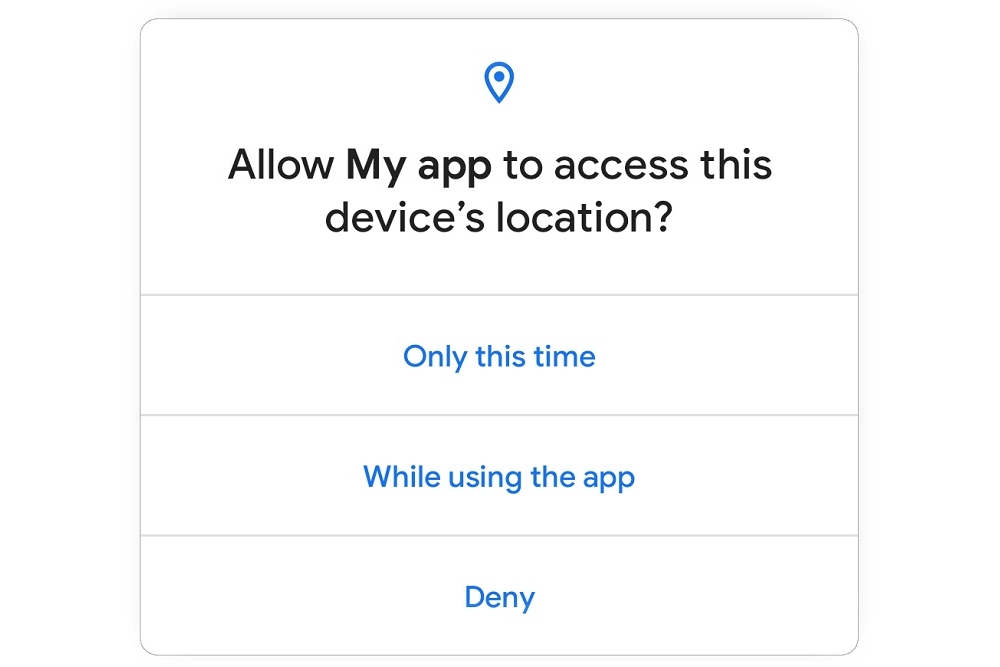The screenshot depicts a permissions prompt from the application "MyApp," which is requesting access to the device's location. The top portion of the prompt features a blue location icon, reminiscent of the one used in Google Maps. Directly beneath the icon, the application's name "MyApp" is prominently displayed in bold black text. Below this, the message "allow MyApp to access this device's location" is shown in regular black text, emphasizing "MyApp" in bold.

The prompt provides three response options, each enclosed within individual white rectangles with subtly curved edges, mitigating any sharp corners. These options are written in blue lettering:

1. **Only this time**
2. **While using the app**
3. **Deny**

The overall background of the prompt is plain white, accentuating the clean and straightforward design of the interface. This setup indicates that the user must choose how they want "MyApp" to handle location permissions, with clear and accessible choices.